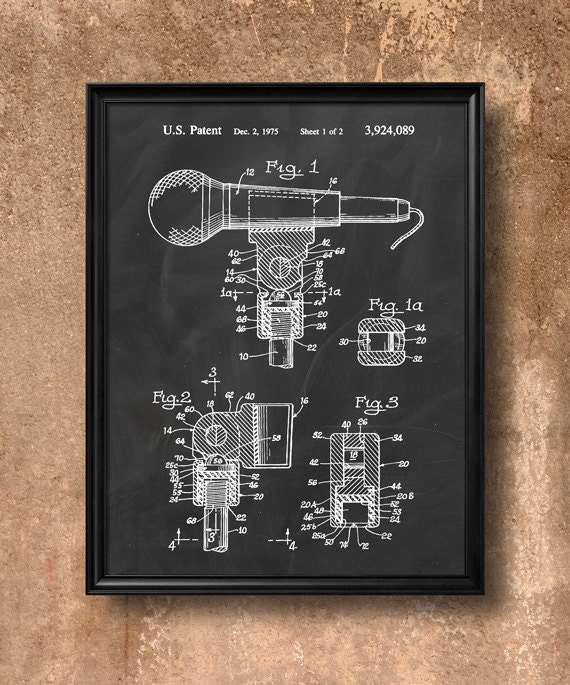This image features a framed patent diagram on a rectangular, black background designed to resemble a chalkboard, complete with wispy white marks. The frame is also black, blending seamlessly with the dark, chalkboard-like background. At the top of the image, it reads "U.S. Patent, December 2, 1975, Sheet 1 of 2, 3,924,089." Central to the diagram is a detailed sketch of a microphone positioned horizontally to the left, with a short length of cord trailing behind it. The microphone is mounted on a stand, and all the components of both the microphone and the stand are meticulously labeled with numbers pointing to different sections. Below the text "Figure 1," various angles of the microphone stand, including top-down and side views, are illustrated, highlighting features such as a pivot mechanism. These additional figures provide a comprehensive visualization of the microphone stand's components and functionality.